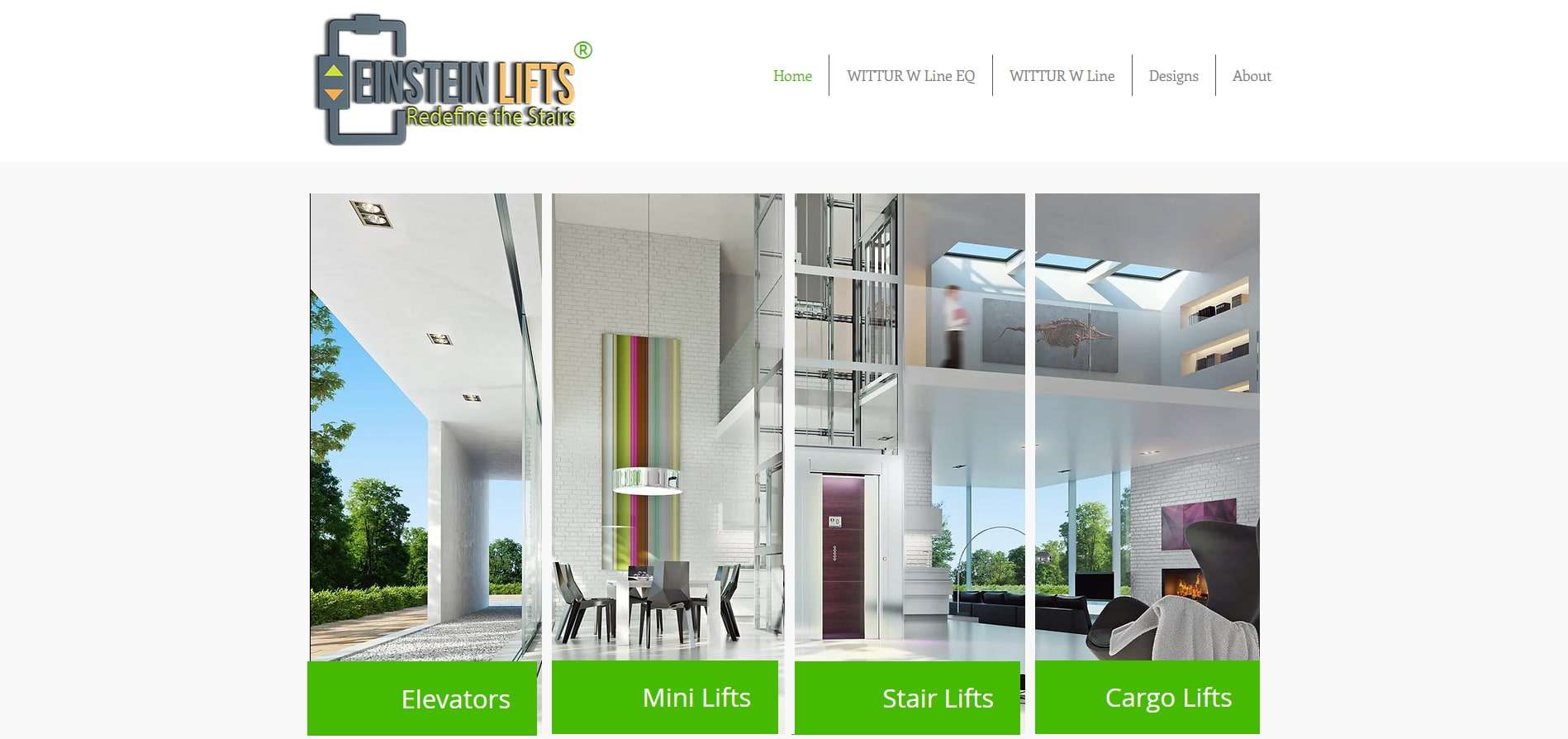The image is titled "Einstein Lifts: Redefine the Stairs." The title presents a novel concept for modernizing staircases, emphasizing innovation in vertical transportation. The text "Einstein" is displayed in gray, while "Lifts" is in orange, with the words compactly arranged without spaces. The name has a registered trademark symbol.

The image includes a simplistic clipart depiction. To the right of a gray board, there is a smaller white box symbolizing an elevator. Below, there's a home button highlighted in green, indicating the current selection. The image is divided into categories by lines, featuring various lift types.

The categories are:

1. **Mini Lifts**: Displayed with a photo of a contemporary architectural entryway with skylights and a traditional rectangular pillar surrounded by trees. The mini lift itself is circular, positioned in front of tables and chairs.

2. **Stair Lifts**: The stair lift is transparent, showing visible cables running vertically.

3. **Cargo Lifts**: Depicted last, illustrating functional designs intended for transporting goods.

Each category is highlighted in a green box with white text. The detailed design elements and listings distinctly showcase the variety and advanced engineering of Einstein Lifts.